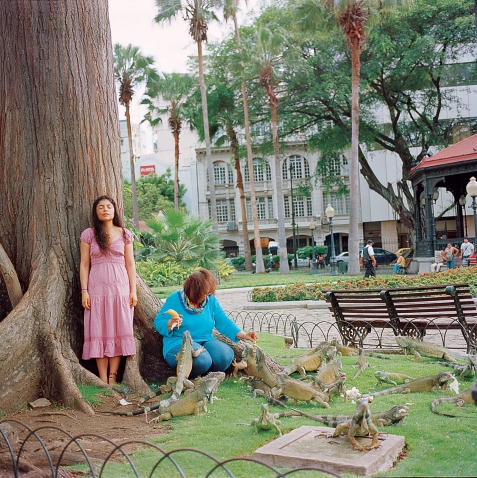In a vibrant outdoor park setting, a young lady in a pink dress with long brown hair and her eyes shut stands serenely in front of a massive tree trunk. Next to her, a larger woman with light brown hair, clad in a turquoise blue sweater and pants, is seated on a root of the tree. She holds a banana in one hand and is feeding a collection of sizeable iguanas gathered in a sectioned-off grassy area enclosed by low arch gates. Behind them, a gray building looms, shaded by palm trees. To the right, a sidewalk bench and a pavilion complete the scene, adding to the tranquil, tropical ambiance.